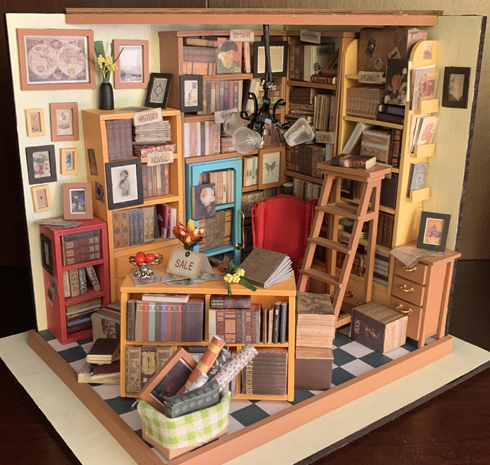This photograph captures an intricately detailed diorama depicting a bustling library or used bookstore scene. The diorama features a black and white checkered floor, partially obscured by an assortment of colorful bookcases—red, orange, blue, yellow, and brown. The back and side walls are lined with bookshelves filled with volumes of books, and art frames with various photographs and artworks interspersed among them. A small wooden ladder leads up to a tall bookcase on the right wall, while another bookcase stands at the forefront, alongside a small basket containing rolls of paper and more frames. The scene includes a plush red upholstered chair and an old-fashioned chandelier hanging above, adding a touch of vintage charm. This miniature room, resembling a library or a used bookstore, is meticulously set on a dark brown lacquered wooden table, creating a striking contrast that highlights the detailed craftsmanship of the diorama.